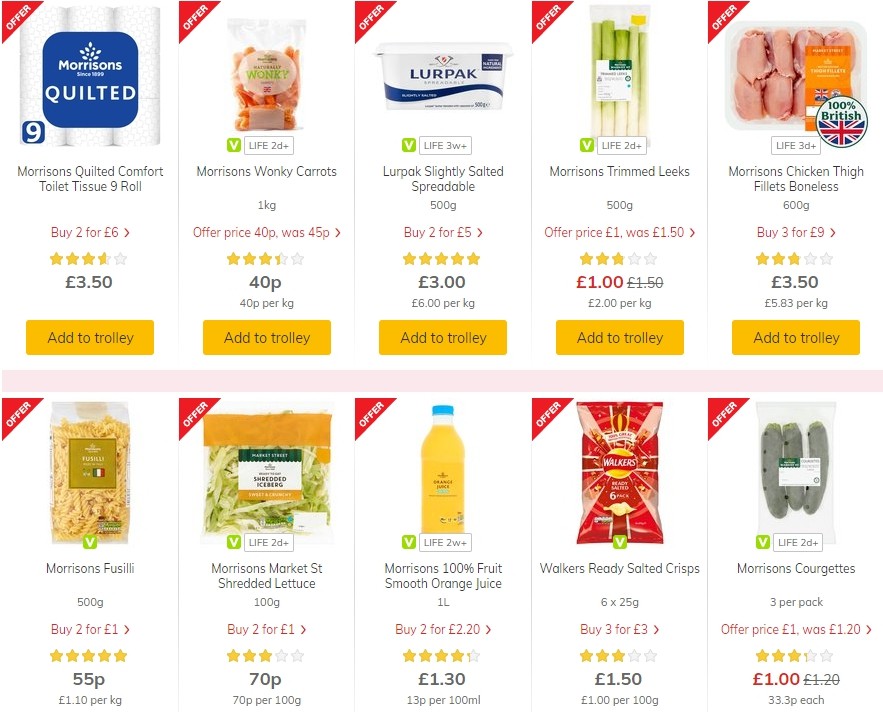A detailed image caption might be formatted as follows:

---

This image is a closely cropped screenshot of a British grocery store’s online shopping platform, likely from Morrisons. Visible are various Morrisons-branded products, reinforcing the store’s identity. The screenshot displays approximately ten items arranged in two rows, comprising basic grocery items. Notable products include Morrisons Chicken Thigh Fillets (boneless), featuring a 100% British sticker, and a button for adding items to the trolley, confirming the British context.

The items displayed include:
- Fusilli pasta
- Shredded lettuce
- Fruit juice
- Walkers crisps (another British brand indicator)
- Morrisons Wonky Carrots
- Morrisons Quilted Comfort Toilet Tissue, in a 9-roll pack
- Lurpak Slightly Spreadable butter, with a shelf life indicator of 3 weeks (3W+)
- Chicken thigh fillets, with a shelf life indicator of 3 days (3D+)

Each product listing includes prices, per kilo costs for food items, shelf life details, and any applicable discounts, providing a comprehensive view of the product offerings and pricing structure.